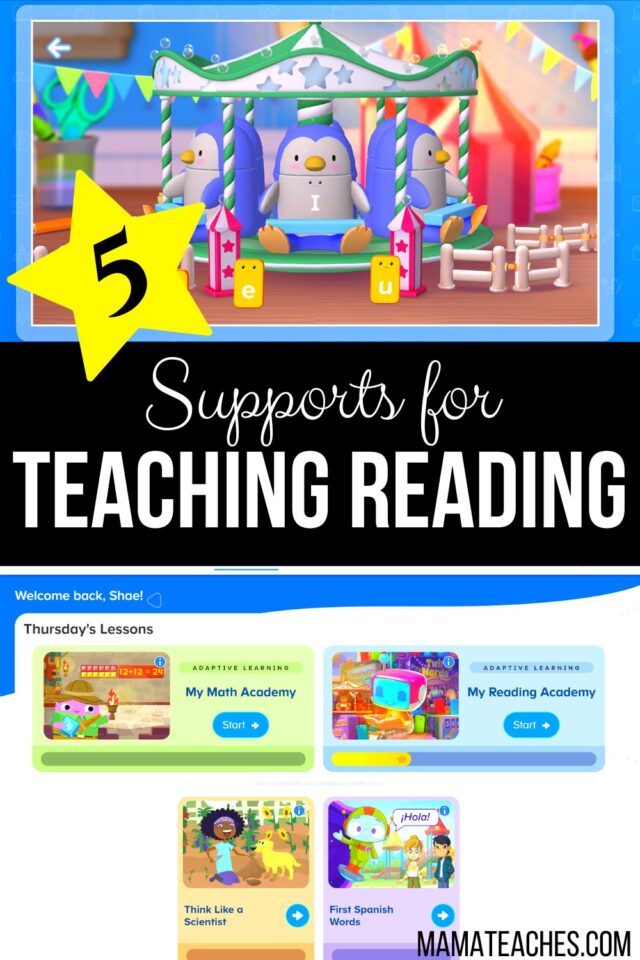This screenshot from MamaTeaches.com features a whimsical and colorful advertisement. In the lower right corner, the website's watermark is visible. The top of the page showcases a carnival scene with charming, cartoon-style penguin characters either forming or riding on a Candy Land-themed merry-go-round. The merry-go-round itself is vibrant and playful, set in a delightful carnival area.

A prominent yellow star with the number five in the center adorns the upper left corner of the page. Just below this, a bold black stripe with white text proclaims, "Supports for Teaching Reading." 

The main content area includes a welcoming message, "Welcome Back, Shoel," indicating a user named Shoel has logged in. The layout features four distinct advertisement boxes each styled in the same Candy Land theme. These boxes list Thursday's lessons: "My Math Academy," "My Reading Academy," "Think Like a Scientist," and "First Spanish Words."